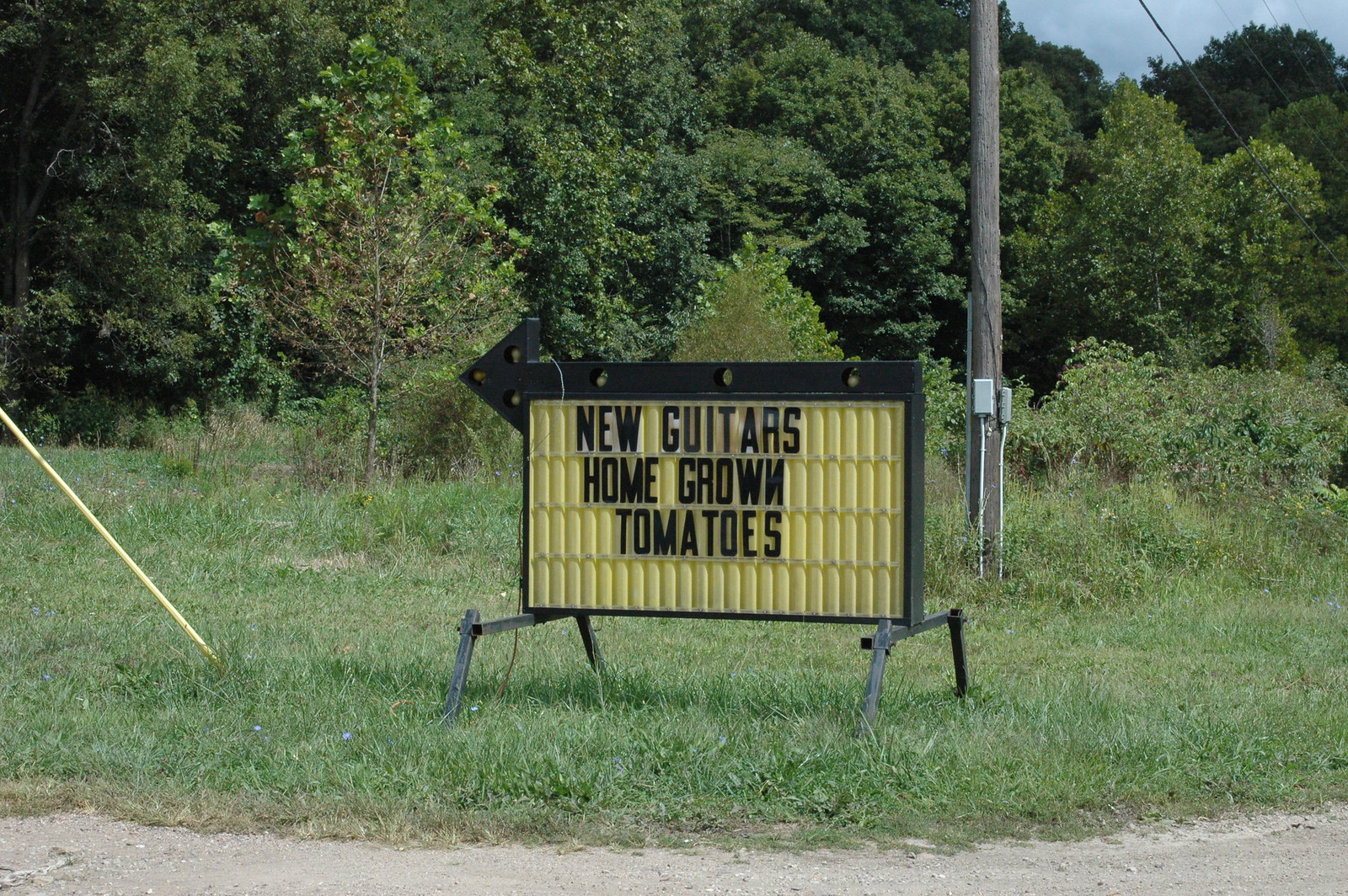This outdoor photograph captures a quaint sign that reads "New Guitars" on the top line, "Homegrown" in the middle, and "Tomatoes" on the bottom line. The text is displayed in a standard black sans-serif font typical of such sign boards. The sign itself is outlined with a black border, which is thicker at the top and features three evenly spaced holes. The structure is mounted on a stand with two supporting legs affixed to the bottom left and right corners, lifting it above the grassy field it stands in.

The background reveals a serene natural setting with an array of trees and a dense forest, creating a lush green backdrop. Closer to the viewer, a telephone pole punctuates the scene, adding a rustic element. The very bottom of the image shows a gravelly dirt path, hinting at a rural or suburban environment rather than an urban one. The overall ambiance of the photo is pastoral and tranquil, blending elements of nature and quaint signage.